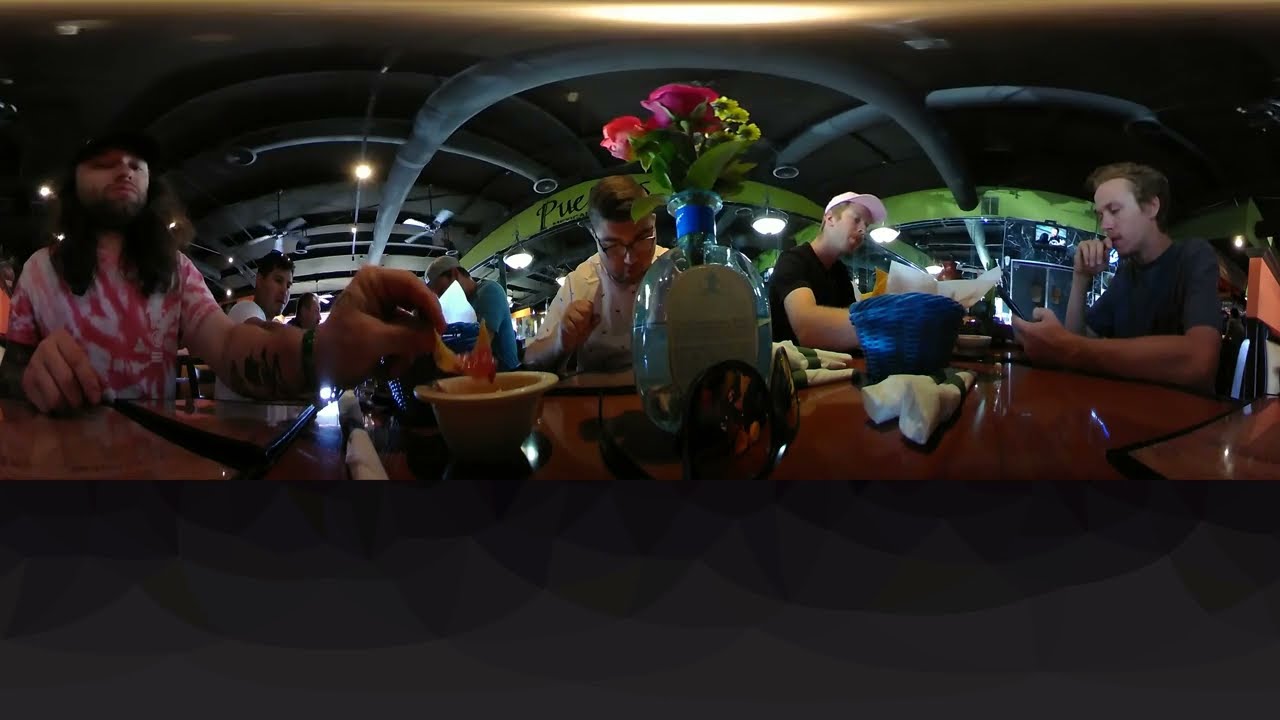The photograph captures a lively scene of people sitting at a wooden table in a casual restaurant bar with a warm, summery atmosphere. The image is slightly warped due to its 360-degree nature, adding a unique perspective. Dominating the left side, a man with a beard, wearing a pink and white tie-dye shirt, hat, and tattoos, joins another man on the right donning a blue t-shirt and engrossed in his smartphone. At the center of the table, a liquor bottle repurposed as a vase holds a floral arrangement. Surrounding this centerpiece are blue baskets filled with food, interspersed with napkins and silverware.

The setting hints at an unfinished industrial design with exposed silver pipes and a contrasting black ceiling, accented by green lining. Two men in baseball caps in the background reinforce the relaxed, summery vibe. The table is cluttered with various personal items, such as sunglasses and a bowl, while natural daylight brightens the scene. The visible colors range from wooden browns and grays to vibrant blues, greens, pinks, and whites. Above the scene, part of the restaurant's name, "Pueblo," is visible on a banner, partially obscured by a patron’s head, adding a personal touch to the vivid snapshot of everyday life.